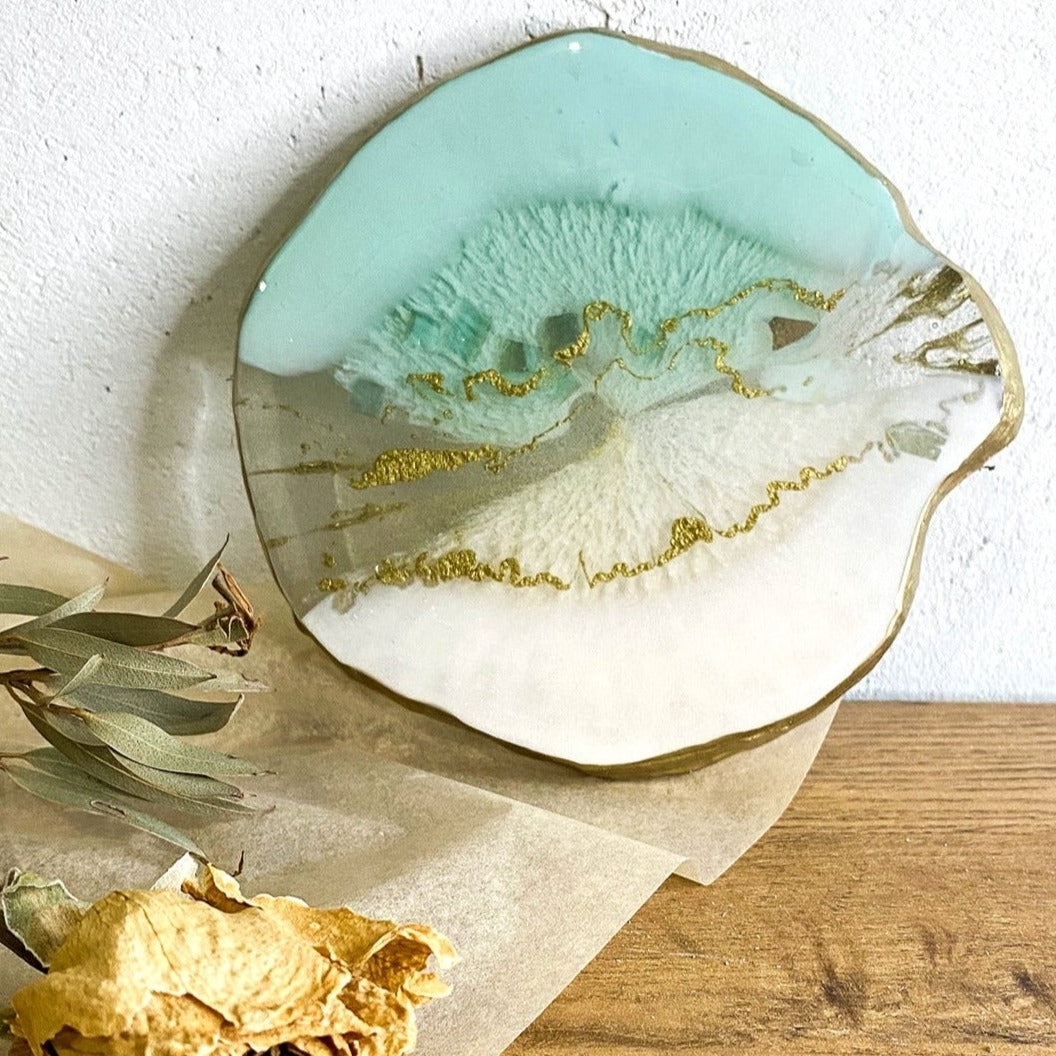The image depicts an intricately decorated, nearly circular piece of wood art, prominently set on a wooden table, resting on what appears to be a piece of parchment paper. The backdrop features a stark white concrete wall, lending contrast to the warm tones of the wood. In the foreground, a few dried plants are artfully placed on the table.

The artwork itself is remarkable, showcasing a blend of materials and colors that create a mesmerizing effect. The outer edge of the piece is adorned with a gold finish, framing the internal design which appears to be sealed with epoxy for a glossy and polished look. The lower half of the artwork boasts a creamy white color, gradually transitioning to a small gray area on the left and then to a light sea foam green-blue shade on the upper half. Swirls of gold are intricately woven through the blue and cream areas, adding a touch of elegance and depth.

Despite some mentions of the artwork resembling rock and glass, the predominant details suggest the use of paint, likely acrylic, with the possible incorporation of other materials to create the varied textures and clear sections likened to stained glass. The overall composition is visually stunning and exudes a beachy, sophisticated charm.